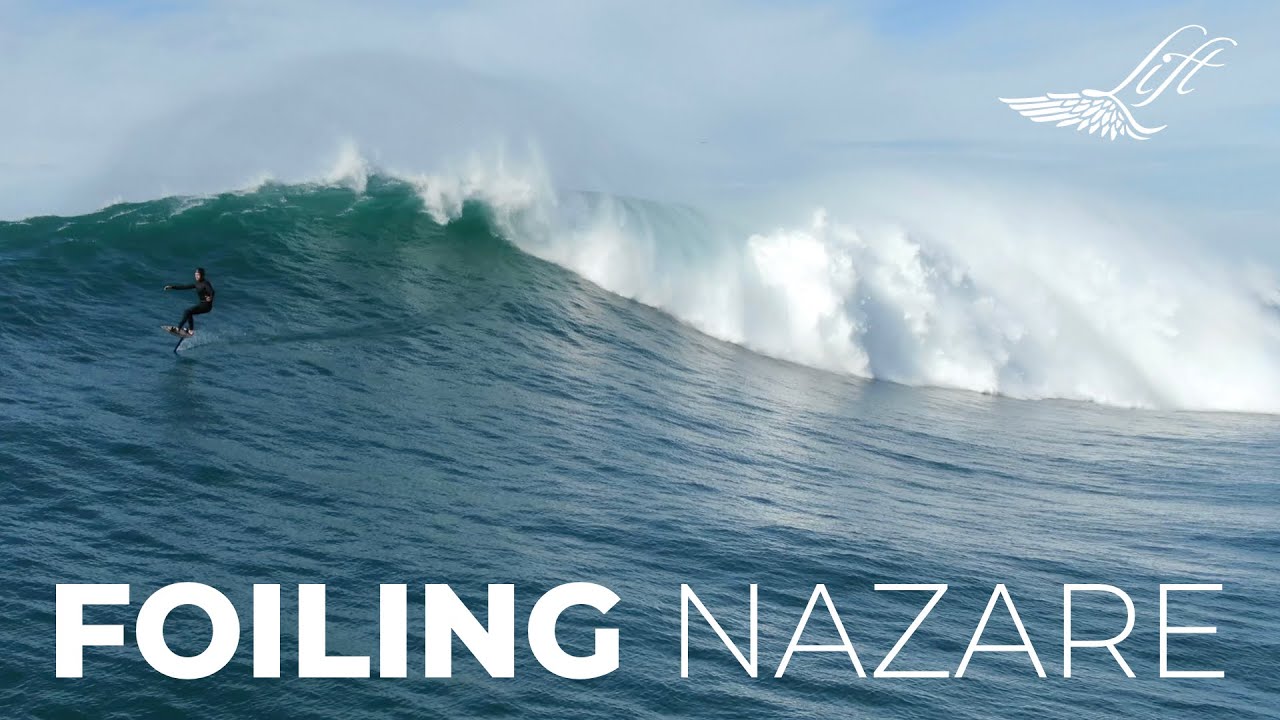The photograph captures a dramatic scene of a large greenish-blue wave, approximately 20 feet tall and 100 feet wide, with a surfer riding its face. The surfer, clad in a full black wetsuit, is positioned on the left side of the image, navigating through the non-foamy part of the wave. In the top right corner, the word "Lift" is elegantly scripted in white with a wing-like graphic beneath it, suggesting a sense of elevation. Along the bottom of the image, bold white text reads "Foiling Nazare," indicating the location in Portugal famed for its enormous waves. The wave crests and crashes on the right, creating a frothy white foam, while the water closer to the camera shifts from green to a deeper blue, set against a backdrop of blue sky scattered with white clouds. The image is a horizontal rectangle, capturing the vastness and power of the ocean with the small, yet daring figure of the surfer adding a sense of scale and human endeavor.